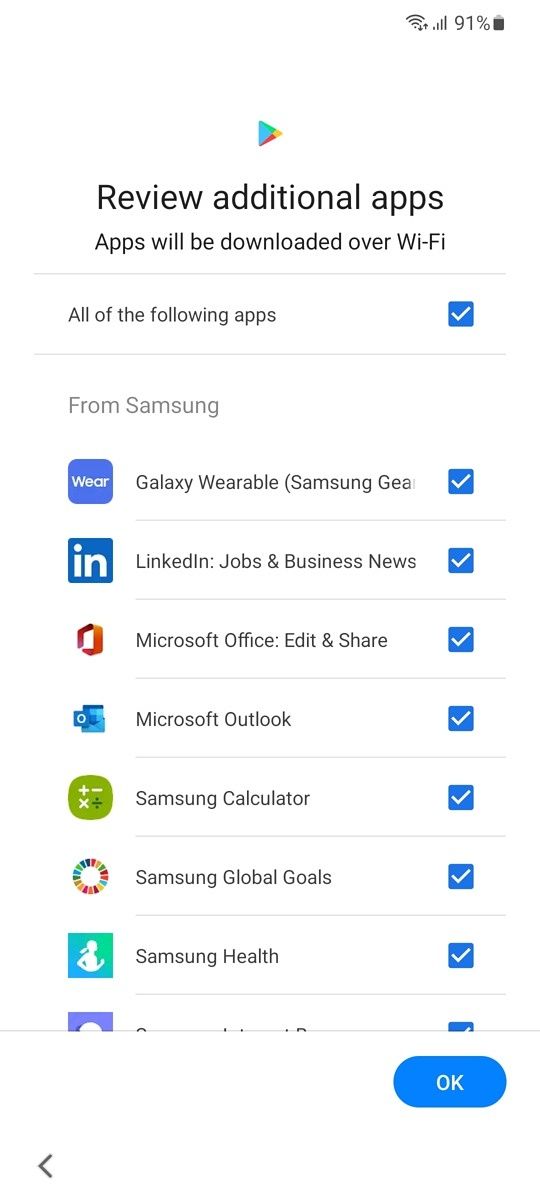A cell phone image captures a screen displaying an app installation process. At the top, there's a heading titled "Review Additional Apps," accompanied by a notification that the apps will be downloaded over Wi-Fi. Below, a list of check-marked apps follows, indicating their selection for installation. 

The first section reads:
- "From Samsung," which includes:
  - Galaxy Wearable
  - Samsung Gear
  - LinkedIn (Jobs, Business News)
  - Microsoft Office (Edit and Share)
  - Microsoft Outlook
  - Samsung Calculator
  - Samsung Global Goals
  - Samsung Health (partially visible but checked)

Each item on the list is accompanied by its respective icon on the left: for example, LinkedIn's distinctive "in" logo and the Galaxy Wearable icon. At the bottom of the screen, a blue "OK" button with white text is prominently displayed, allowing the user to proceed with the installations.